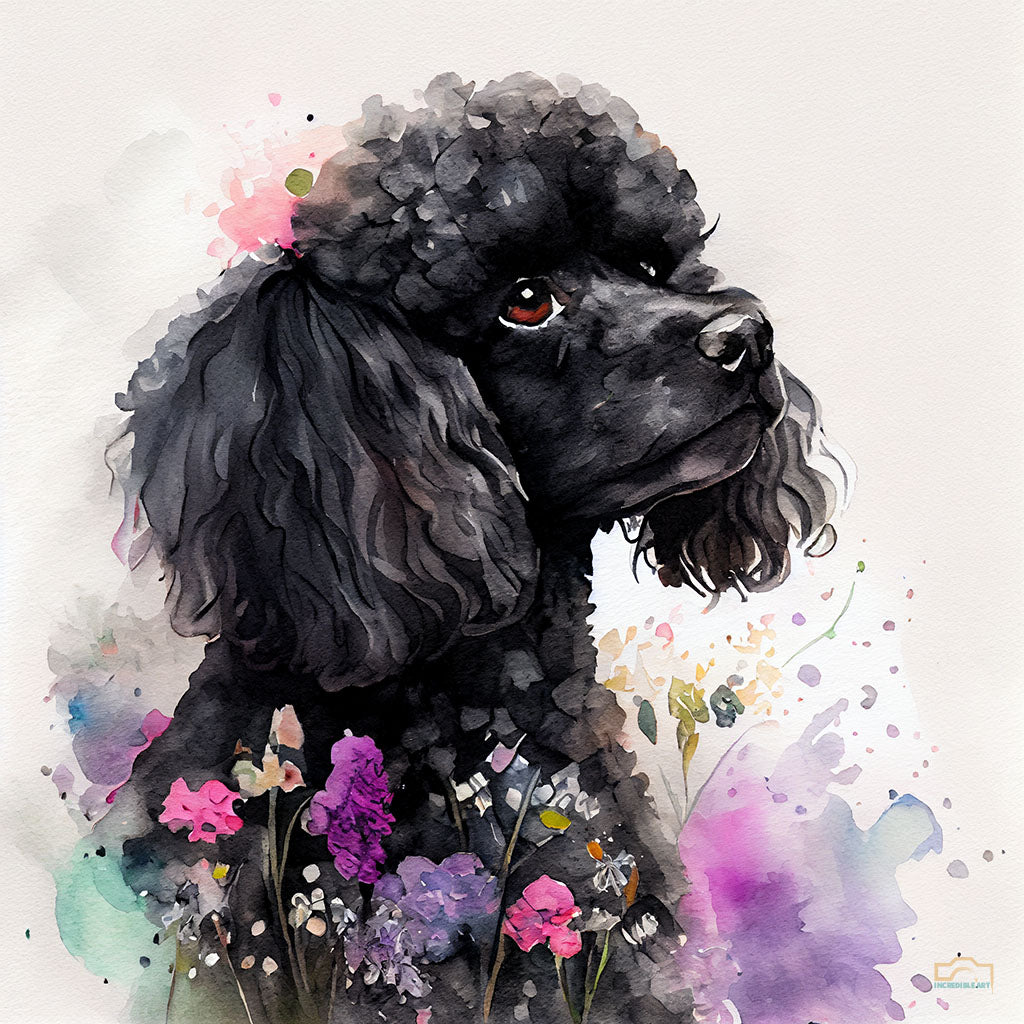The image is a square watercolor painting, approximately five to six inches in height and width, featuring a black poodle. The poodle, with its curly poof of fur atop its head and fluffy, rounded ears, appears from the lower right corner, facing right. Its dark brown eyes look upward, creating an engaging profile. The painting's background is a textured off-white with a slight brown or yellowish tint, providing a neutral canvas for the main subject. Surrounding the dog are vibrant flowers in shades of pink, purple, and peach, accompanied by splashes of light blue, adding a lively contrast to the composition. There are additional colorful paint splashes around the bottom of the picture, enhancing the abstract feel of the artwork. A watermark, reading "incredible art" in blue print, is located in the lower right corner, although another source suggests it might be in the bottom left corner but hard to read due to resolution.